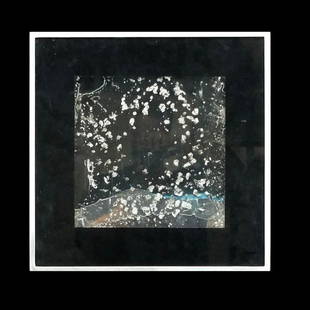The image appears to be an abstract piece of artwork with a layered, minimalist composition. It features a perfectly black outer square functioning as a frame, followed by a skinny white border. Within this, there's a thicker, textured black border. Inside this black border lies the main area of the artwork, which is predominantly dark gray with shimmering effects and varied textures. Strewn across this central area are numerous randomly-placed white splotches, reminiscent of flower petals or rock-like speckles. Towards the bottom, these white splotches seem to merge with a lighter, watered-down streak of paint, introducing subtle hints of brown, blue, gray, and possibly a touch of green. This layered, textural interplay of colors and shapes creates a visually intriguing and complex piece, though it's ambiguous whether it is the work of a professional or an amateur artist, as there is no text or signature to provide further context.